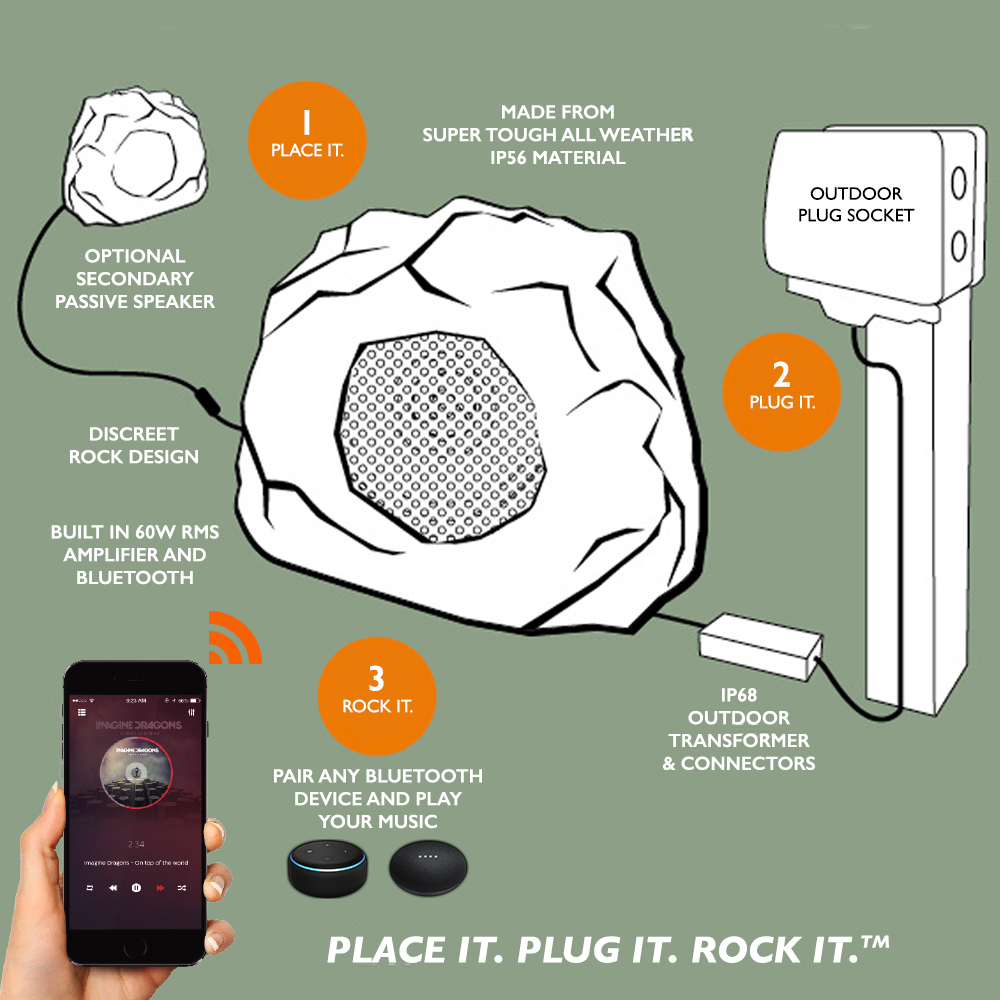The advertisement showcases a square, six-inch by six-inch diagram set against a grayish-green background. At the top center, bold white text reads, "Made from SuperTuff all-weather IP56 material." Central to the image is a white, rock-like object with a mesh center, representing a speaker. To its right, another white object labeled "outdoor plug socket" is shown, with a long, rectangular stand. A wire connects this socket to a second white rectangular shape, described as an IP68 outdoor transformer and connectors. To the left of the main speaker is an illustration of an optional secondary passive speaker, similarly designed as a rock. Both rock speakers feature a built-in 60W RMS amplifier and Bluetooth capability, allowing users to pair any Bluetooth device for music playback. In the lower left corner, a Caucasian woman's hand holds a cell phone displaying "Imagine Dragons" with an orange sound bar. Bold white text at the bottom of the image reads the slogan: "Place it. Plug it. Rock it." An orange circle with a white number indicates steps: 1. Place it – position the speaker, 2. Plug it – connect to the outdoor socket, and 3. Rock it – play your music.